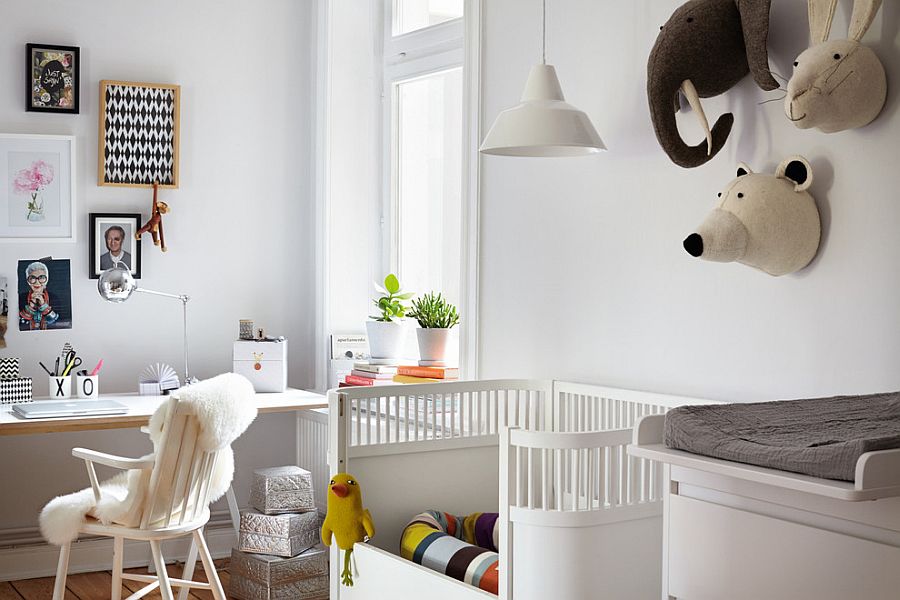This high-definition color photograph captures a modern, multifunctional baby's room and office bathed in bright natural light. Dominated by white walls and warm wood flooring, the room is accented with splashes of color. On the left, a baby’s crib with a multicolored striped bedspread holds a plush yellow duck toy. Adjacent to the crib is a white changing table topped with a gray cover. Above this area, plush heads of a bear, a rabbit, and an elephant are mounted on the wall. Hanging from the ceiling, a pendant light illuminates the space.

In the center, a large window with white curtains floods the room with light. Two green potted plants sit on stacks of books on the windowsill, adding a touch of nature to the room. To the right, a white desk equipped with office supplies, a laptop, and containers holding pens stands beneath wall-mounted pictures of famous people and colorful artworks. Below the desk, three silver boxes provide additional storage. A white chair draped with a faux fur throw completes the setup, making it a practical workspace for a parent to attend to both office duties and baby care seamlessly.